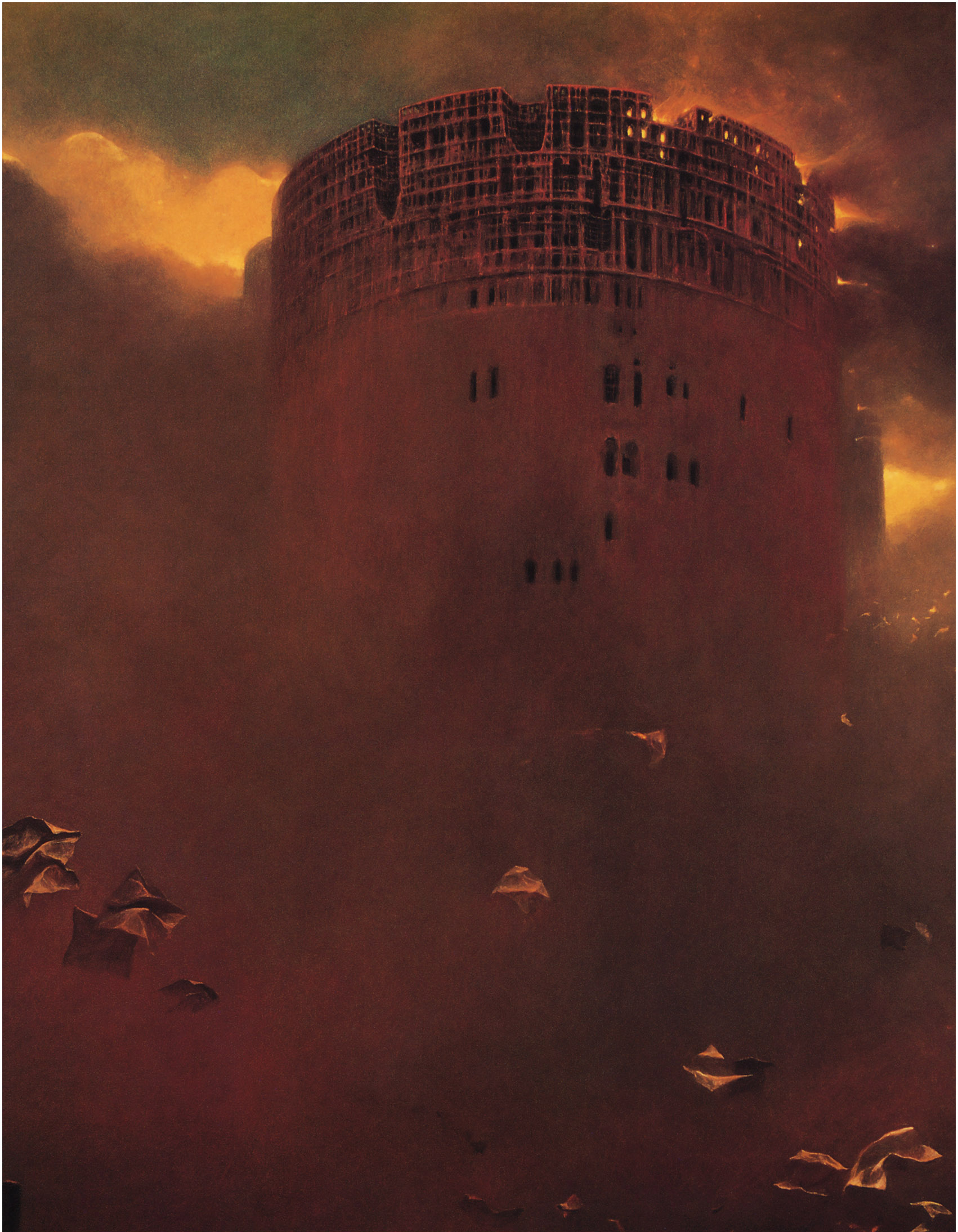This artwork is a painting of a towering, cylindrical structure set against a dramatic outdoor sunset at night. The top half of the tower appears incomplete, revealing skeletal, framework-like ruins with exposed beams and multiple dark, black windows. The structure evokes the appearance of a coliseum, with its round shape and multi-storied height. The backdrop is an arresting blend of deep reds, purples, and grays, giving the scene a smoky or dusty atmosphere. Hints of bright, orange sunlight peek through dark clouds at the top, casting a haunting, ethereal glow over the scene. Below, the middle and bottom parts of the image are enveloped in darkness, punctuated by a series of white triangular shapes resembling tents scattered in a field, accentuated by fine highlights of white and black.